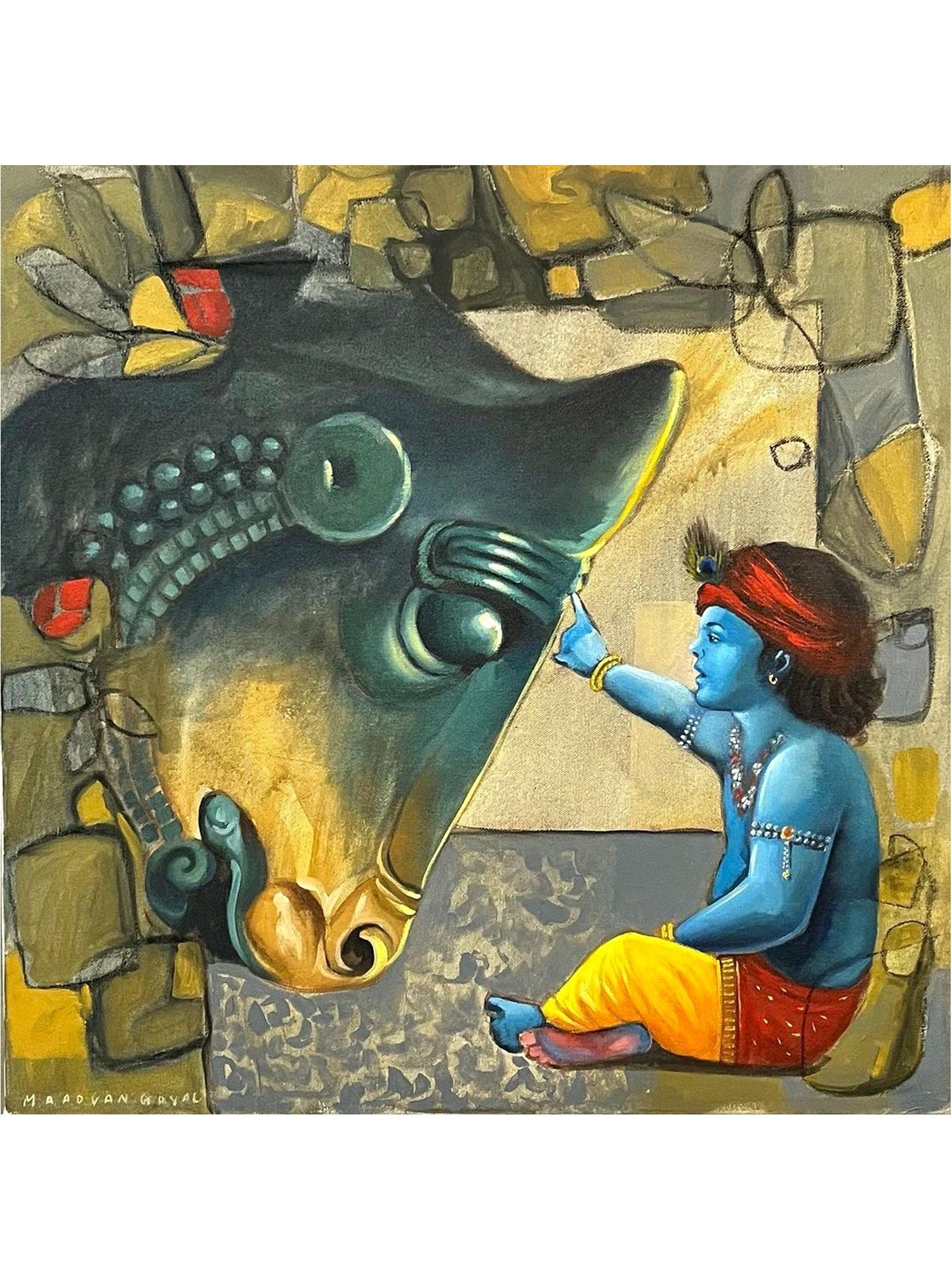The image depicts a detailed, culturally significant artwork, possibly inspired by Hindu mythology or Indian folklore. In the lower right quadrant, there is a miniature blue-skinned person, likely representing a deity or mythological figure, seated cross-legged. This figure, seen in profile facing left, has shoulder-length dark hair adorned with a red turban featuring a small feather at the front. They are embellished with jewelry, including gold bands on their upper arms and wrists. The figure wears distinctive pants that are red around the waist and yellow down the legs.

The scene is set against the backdrop of a stone archway that stretches above and to the left of the figure. This arch suggests a cave-like structure made of gray and yellow bricks. The blue figure extends their right arm towards a large, ornate head of a bovine or equine statue positioned within the archway. This statue, possibly representing a horse or bull, is adorned with rings on its forehead and a beaded ornamentation along the side of its head. The statue's head, primarily black with yellow accents around the nose and mouth, appears to be bowing down as it connects with the figure's outstretched pinky finger. In the bottom left corner of the image, there is a faint watermark in small yellowish-white font, which is difficult to read due to its size.